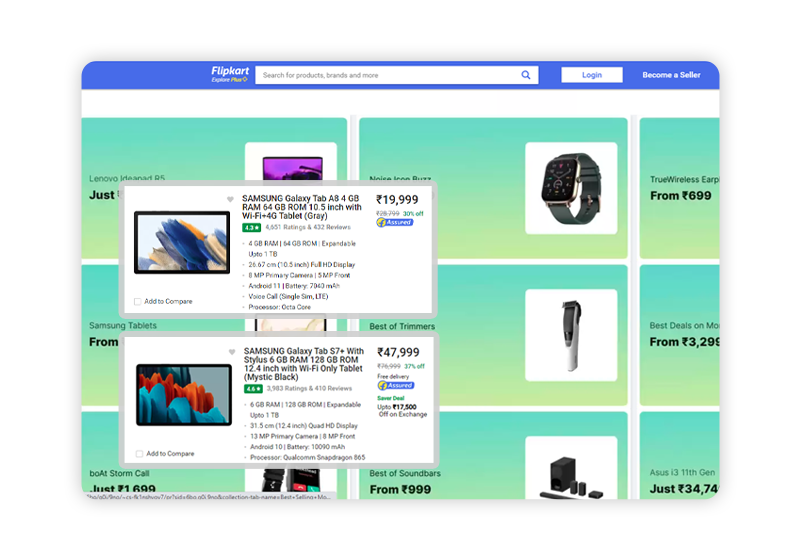The image depicts an online shopping platform with a prominent blue header labeled "Flipkart." At the top of the page, there is a search bar for users to find products. A white rectangular button in the header is labeled "Login" in blue text. Below the header, the page's main content features a clean white background showcasing six rectangular sections, each dedicated to different technology devices.

In one of these sections, there is an image and description of a Samsung Galaxy Tab A8 tablet. This tablet offers 4GB of RAM, 64GB of storage, a 10.5-inch screen, and is equipped with both Wi-Fi and 4G capabilities. The tablet image is encased in a white rectangle, and its price is listed as ₹19,999. The price is accompanied by a checkbox labeled "Add to compare."

Another section on the page features the Samsung Galaxy Tab S7 Plus, which includes a stylus. This model boasts 6GB of RAM, 128GB of storage, and a 12.4-inch screen, but is limited to Wi-Fi connectivity. The tablet, described as "Mystic Black," is priced at ₹47,999 and also has a checkbox labeled "Add to compare."